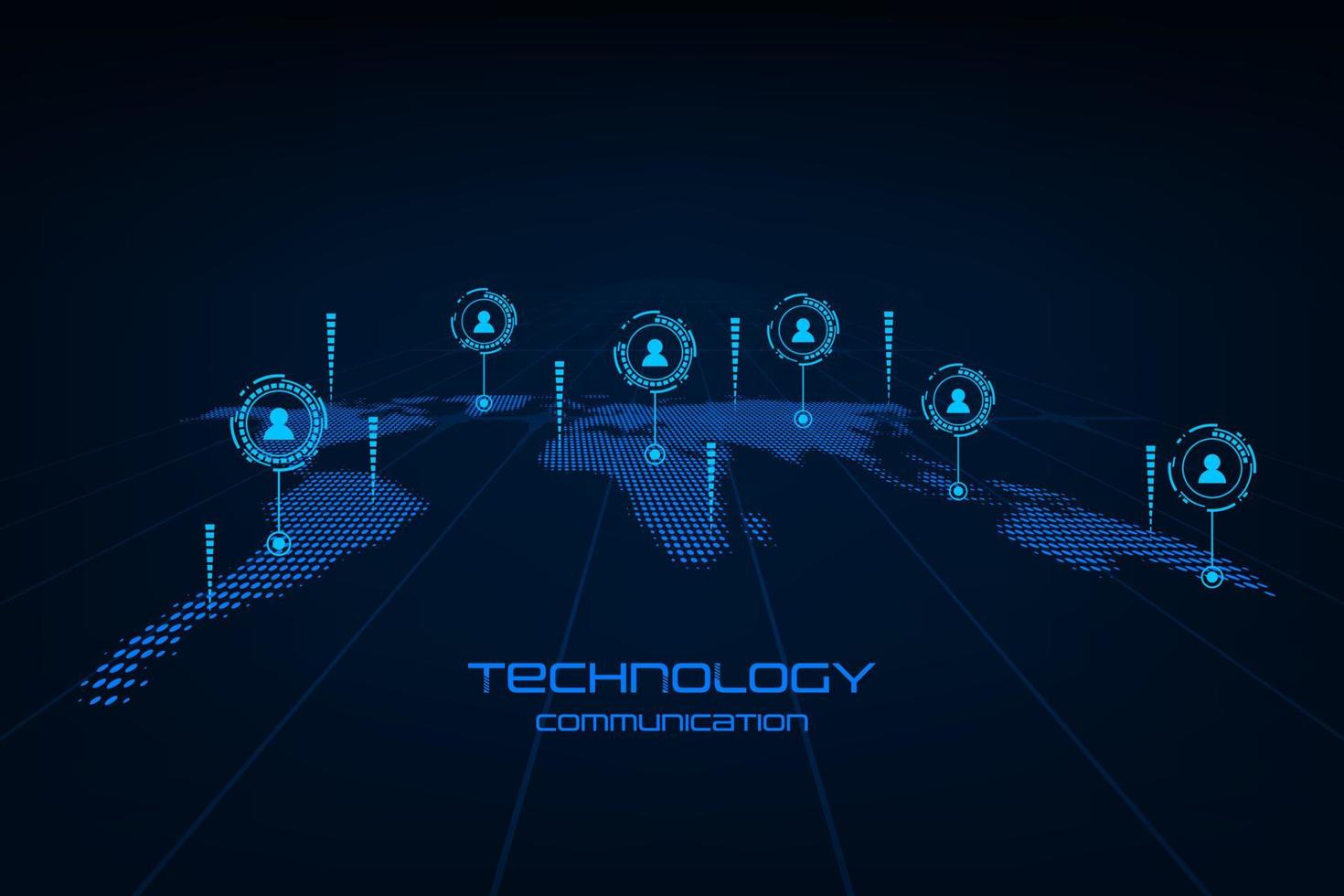The image is a computer-generated graphic with a predominantly dark blue background. It features a world map, illustrated in dots, with a slightly tilted, 3D appearance that highlights continents such as North America, South America, Africa, Europe, Asia, and Australia. At the bottom, the map is superimposed on a grid with lines extending across. Various blue bars rise from specific locations on the map, and a circular display with a person's face, possibly indicating different loading capabilities or communication nodes, is also visible. Six circles containing silhouettes of a stick figure's head and shoulders are positioned above various continents. The text "TECHNOLOGY COMMUNICATION" is prominently displayed in capital light blue letters at the bottom of the image.